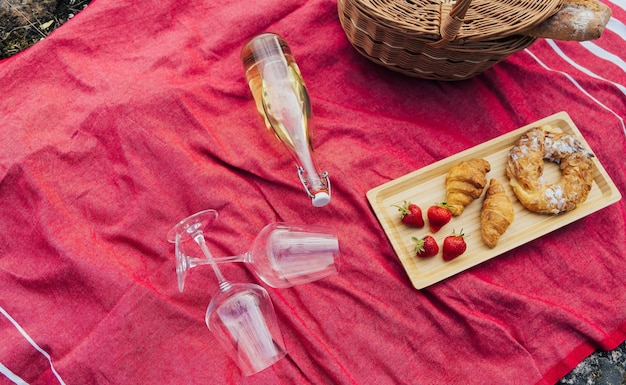This detailed photograph captures a tranquil picnic scene from an aerial perspective. A red, wrinkled blanket with white stripes at either end is spread out on the grass, serving as the base for the picnic setup. At the center, there is a wooden tray displaying an arrangement of four ripe strawberries, two golden croissants, and a circular pastry akin to a Danish. Beside this, two empty wine glasses lie on their sides with their stems crossing, complemented by a bottle, possibly white wine, positioned horizontally nearby. The upper right corner of the image reveals a partially visible woven wicker basket, with a loaf of bread peeking out. The entire setup exudes a serene and appetizing atmosphere, making the scene appear inviting and idyllic.